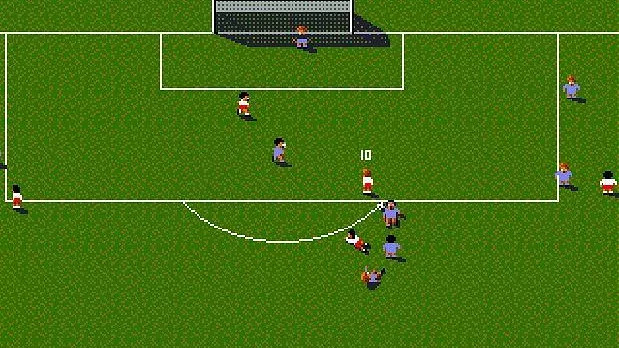In this image, we see a dynamic soccer scene displayed on a video screen. Two teams are engaged in a critical moment near the penalty zone, with one team donning red shorts and white tops, and the other team clad entirely in blue. The players are clustered just inside the arc, suggesting a tense situation possibly leading to a penalty shot. The ball's exact location is not clear, but there is an indicator showing the number "10" above one of the players, which might refer to points or player number. The goal is visible in the background, and it appears that the goalkeeper, wearing a distinct outfit, is prepared for action. The green field serves as the backdrop, which is encircled by various on-screen graphics, including boxes and circles for a detailed overview. Both teams seem evenly matched in numbers, with six players each, including their respective goalkeepers. There is also a hint that the ball might be placed on the penalty circle, particularly towards the top right edge of the image.